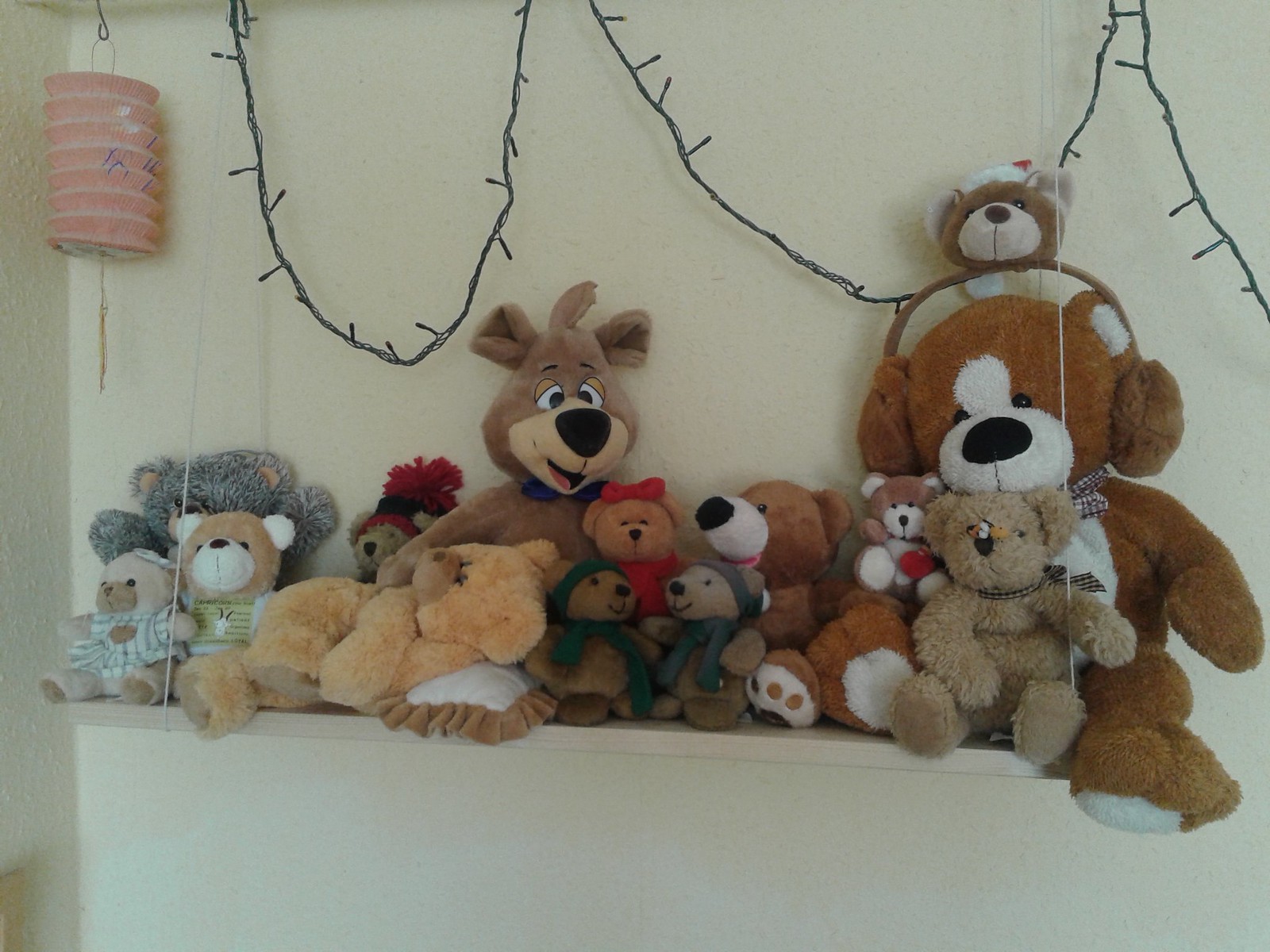In this image, a variety of animal plush toys, predominantly teddy bears, are neatly arranged on a light wood shelf against a textured, cream-colored wall. There are approximately 14 to 15 bears sitting along the shelf, displaying a range of colors from light tan and medium brown to gray. The bears are adorned with various accessories, including hats, earmuffs, bows on their heads and around their necks, scarves, and shirts. The shelf is decorated with strings of colorful Christmas lights draping down from above, and in the upper left-hand corner of the image, a light red-orange lantern-style fan adds an oriental touch. The bears vary in size, with some being very small and one notably larger bear wearing earmuffs and holding a small bear on top. Gray string lights also hang across the upper third of the scene, enhancing the festive atmosphere.